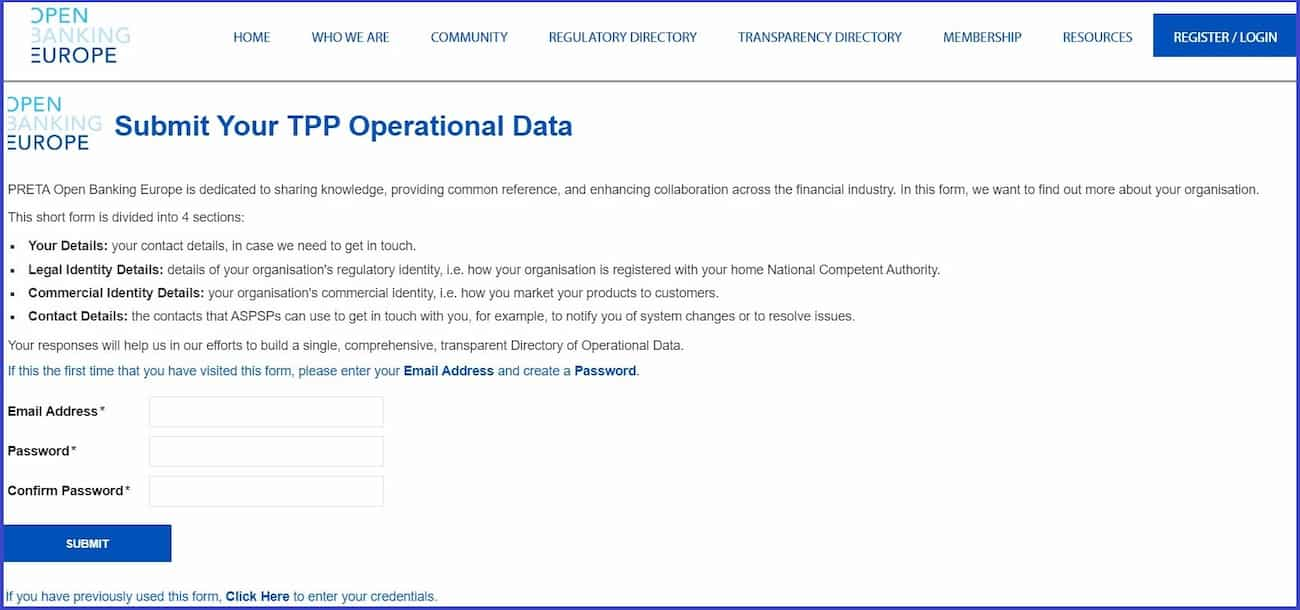The image displays a webpage with a white banner at the top, featuring a collection of blue text. In the upper left corner, the logo "Open Banking Europe" is prominently visible, with "Open" in baby blue, "Banking" in gray, and "Europe" in navy blue. This likely represents the site name or logo.

Below the banner, a navigation menu includes buttons for Home, Who Are We, Community, Regulatory Directory, Transparency Directory, Membership, Resources, and a blue Register/Login button.

The main content area of the page presents a call to action: "Submit your TPP operational data." It emphasizes that Open Banking Europe is committed to sharing knowledge, providing common references, and enhancing collaboration across the financial industry. The form on this page aims to gather more information about participating organizations and is divided into four sections:

1. **Your Details**: Basic information about your organization.
2. **Contact Details**: Information for potential follow-up.
3. **Legal Identity Details**: Details about your organization's registration with the home national competent authority.
4. **Commercial Identity Details**: Details on how your organization markets its products to customers.
5. **Contact Details**: Points of contact for ASPSPs (Account Servicing Payment Service Providers) to notify about system changes or to resolve issues.

The responses will contribute to building a comprehensive and transparent directory of operational data. First-time visitors are prompted to enter their email address and create a password. Below this prompt, there are fields for Email Address, Password, Confirm Password, and a blue Submit button.